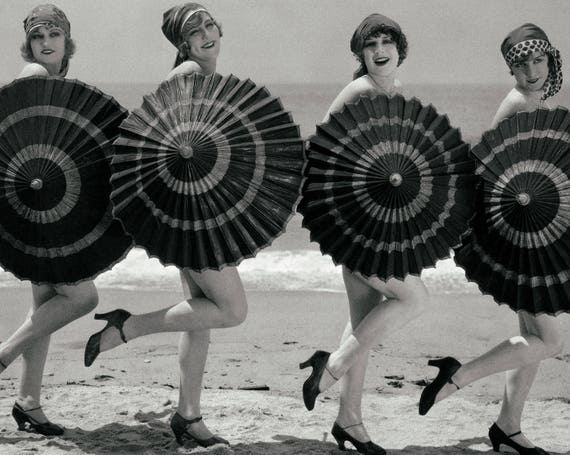This black-and-white photograph, evocative of the 1930s flapper era, captures four women standing in a line on a sandy beach, with the ocean and beautiful sky in the background. The women, resembling showgirls or dancers, strike a coordinated pose with their bodies facing right and their gaze directed towards the camera, each smiling. They hold open parasols that extend sideways from left to right, cleverly concealing their bodies and suggesting nudity beneath. The parasols, possibly made of paper mache, feature intricate designs with two concentric rings that draw the viewer's eye. Each woman wears high heels with straps, likely around four inches high, and their right legs are bent at a graceful 45-degree angle, giving the appearance of a dance move. Complementing their stylish appearance, they have head wrap scarves—reminiscent of flapper bonnets—covering their hair, the length of which is cut just above the shoulders. The women’s makeup, although depicted in grayscale, vividly implies the bold era-specific aesthetic of cherry red lipstick and dark eyeliner. The incoming tide suggests they are quite close to the water's edge.